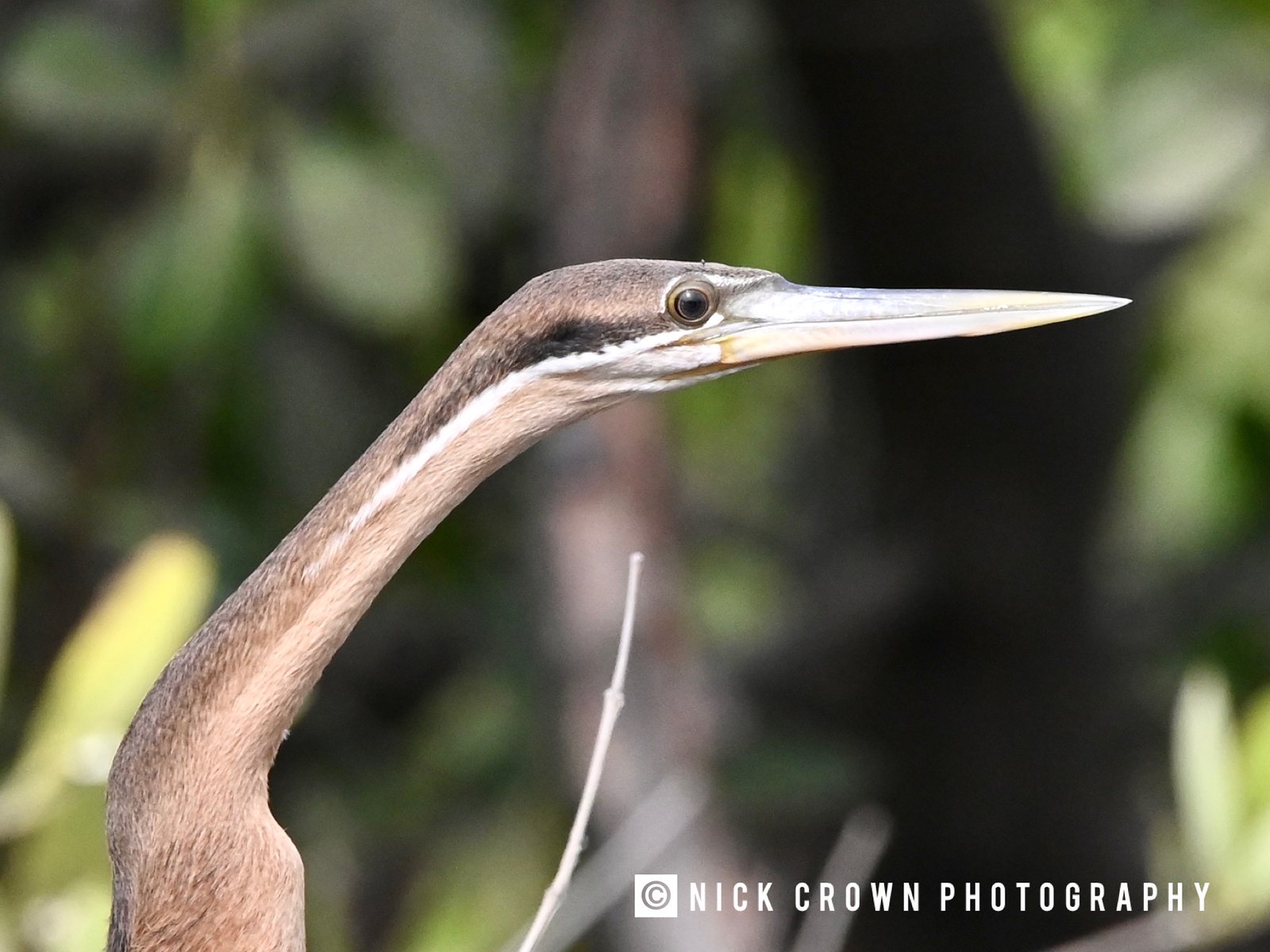This full-color advertisement for Nick Crown Photography features a striking outdoor image captured in what appears to be a wilderness setting. The centerpiece of the photograph is a bird, likely a heron or an African darter, distinguished by its very long, slim neck and unusually lengthy, light-colored beak, tinged with a hint of orange near the base. The bird is shown in a sharp side profile, facing right, allowing a clear view of its intricate feather details, particularly around its neck and head. Its coloration is primarily a mix of brown, gray, and white, with a large, dark eye adding to its distinctive look. The background is a blur of green leaves and branches, suggesting a natural and possibly tropical or southern habitat, captured during the daytime. At the bottom right corner, the text "Nick Crown Photography" in all uppercase white letters, accompanied by a small copyright symbol, subtly identifies the artist, blending seamlessly with the minimalist yet evocative nature of the photograph.